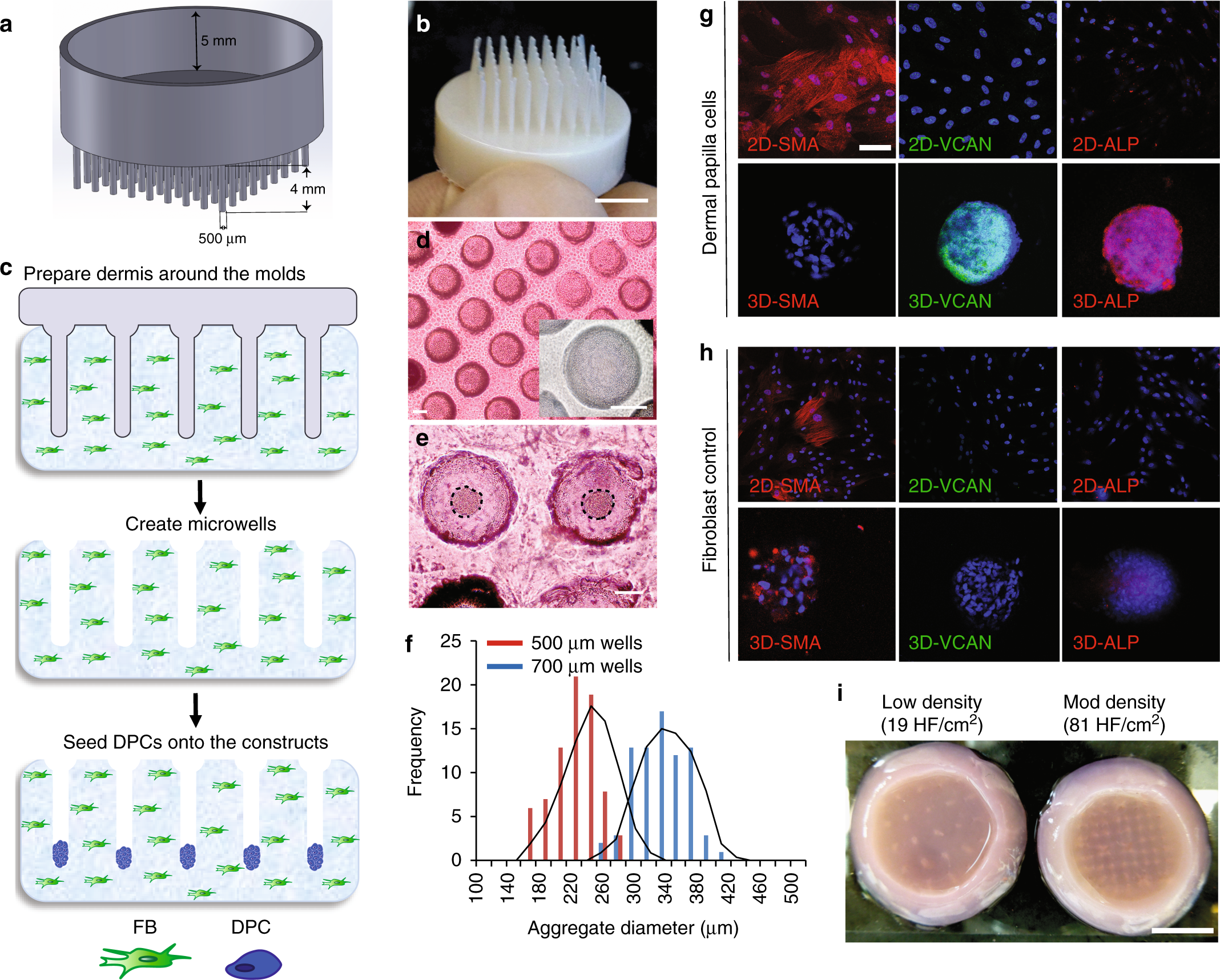This scientific illustration, seemingly drawn from a textbook or scientific manual, depicts a multi-step procedure for preparing and utilizing molds to grow living organisms, particularly focusing on cell cultures. The illustration is divided into several labeled sections, A through J, with each section representing a distinct part of the process.

- **Label A**: Shows a round, circular gray mold with measurements indicating it is 5 millimeters by 4 millimeters. Several tubes are visible coming out from the bottom.
- **Label B**: Depicts a similar object to Label A, but in white plastic instead of metal.
- **Label C**: Outlines three steps for "preparing the dermis around the molds," hinting at some skin involvement.
- **Label D**: Close-up images, possibly taken through a microscope, show the creation of microwells.
- **Label E**: Demonstrates the seeding of Dermal Papilla Cells (DPCs) onto the constructs, with detailed images of cell cultures.
- **Label F and G**: Various colored scans showing different phases or types of cellular growth.
- **Label H**: Presents dark colored scans grouped in two rows of three, possibly assessing the formation or density of micro wells.
- **Label I**: Displays two slightly peach-colored circular objects, which appear to be sliced open, indicating further preparation of the molds.
- **Label J**: Contains a graph with frequency on one axis and aggregate diameter on the other, likely illustrating data on cell growth or mold structure.

This detailed illustration provides a step-by-step scientific protocol, from mold preparation, through different stages of cell cultivation, all the way to data analysis with graphical representation.